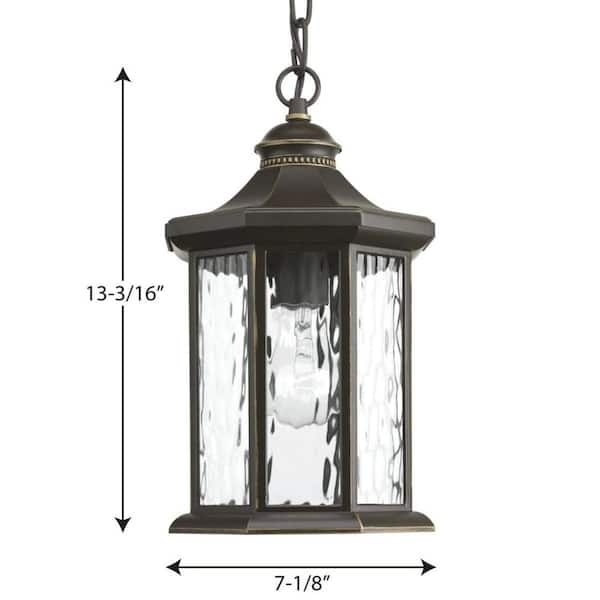This is a detailed photograph of a hexagonal hanging lantern, an image suitable for an Amazon listing or product box for retail sites like Home Depot or Lowe's. The lantern features a dark bronze casing accented with black and gold, containing multiple wavy, textured glass panes. A clear light bulb is visible inside, screwed into the lantern. The design includes a black chain and bracket at the top, allowing it to be suspended from an overhang or ceiling, making it ideal for an entranceway or archway setting. A power cable is wound through the chain, contributing to its functional and decorative appeal. Dimensions are clearly marked on the image with arrows: the height is 13 and 3/16 inches, and its width is 7 and 1/8 inches.